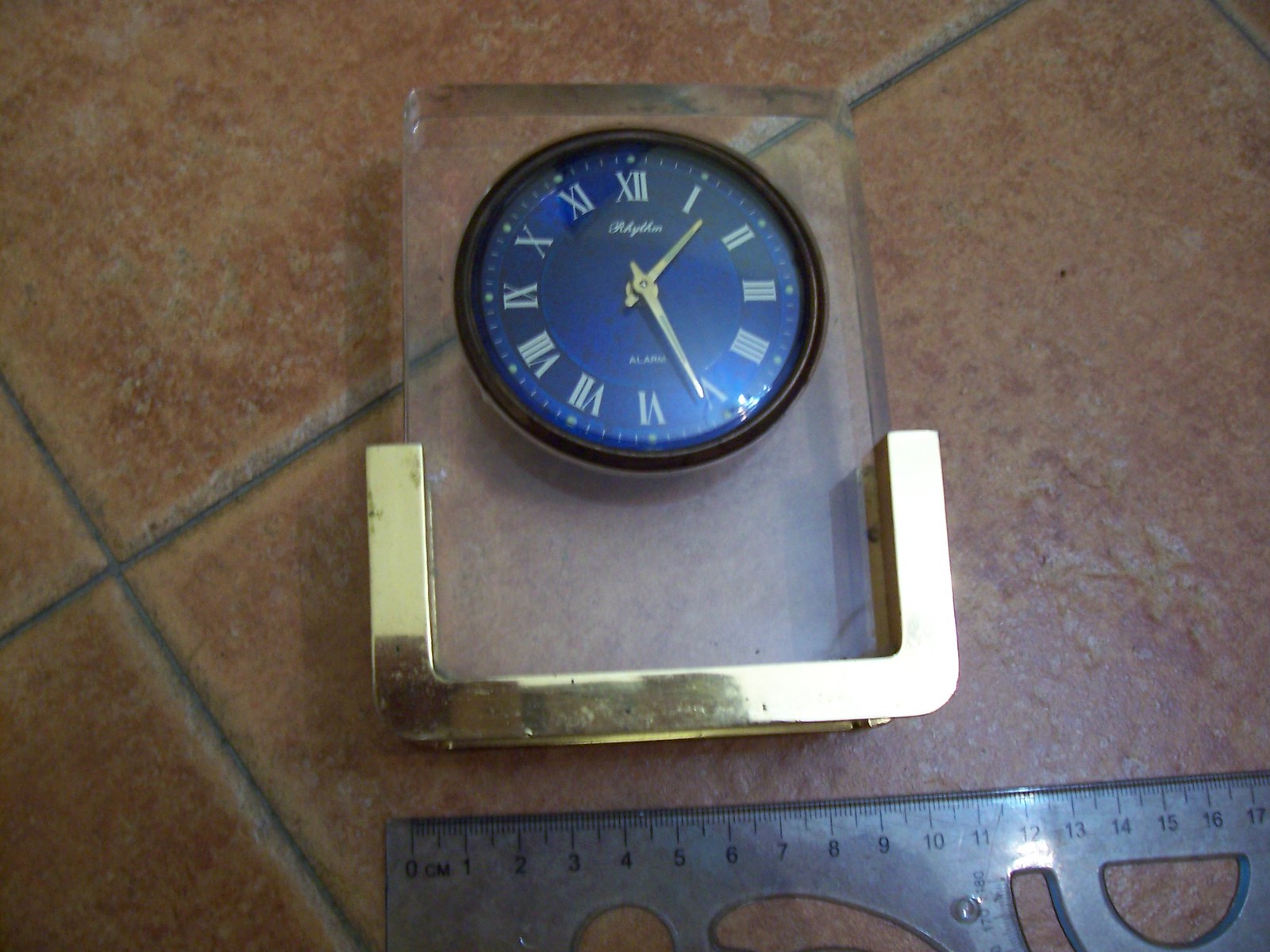The image showcases a detailed, top-down view of a reddish tiled floor with a distinct black line of grouting between the tiles, which form a corner in the bottom left-hand side of the frame. Positioned prominently at the center is a small, intricate clock. This clock features a clear, rectangular vertical body set into a golden, metallic U-shaped base. Embedded within the clear glass is a round clock face that has a dark black border and a blue interior adorned with gold hands and metallic Roman numeral numbers. The face includes white or silver-colored text underneath the Roman numeral 12 in cursive, and additional readable text at the bottom that mentions "alarm." In the lower right-hand corner of the image lies a translucent blue plastic ruler marked in centimeters, displaying measurements from 0 to 17 centimeters with multiple irregularly shaped holes along its length. The clock's width is approximately 11 centimeters when measured against the ruler.